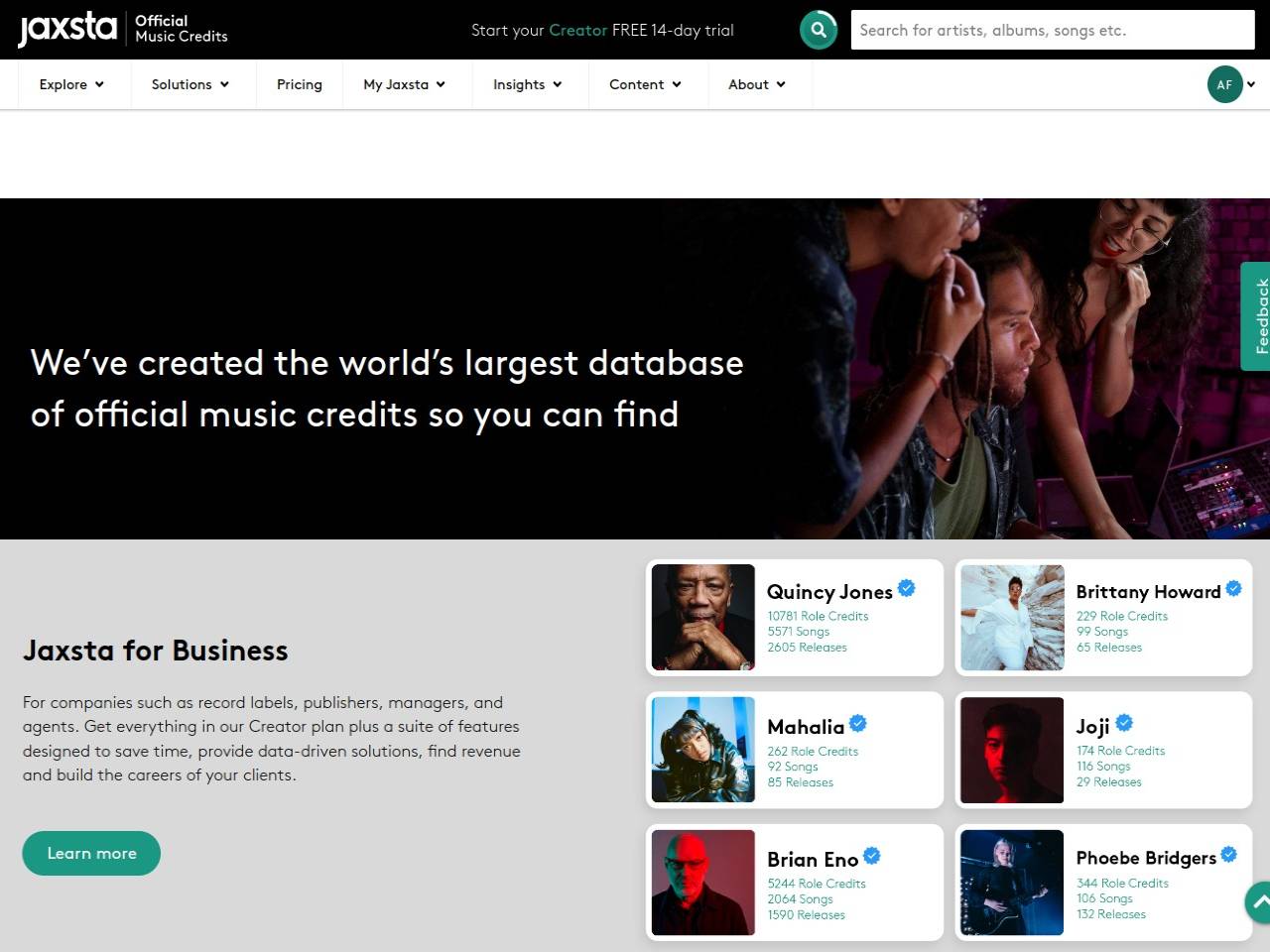The image showcases the homepage of Jaxsta, a website dedicated to Official Music Credits. Dominating the center of the page is a prompt encouraging users to "Start Your Creator Free 14-Day Trial," accompanied by a search icon and a search bar. The input placeholder within the search bar reads, "Search for Artists, Albums, Songs, etc.," in gray text. The background of this section is black.

Directly below this, a white navigation strip spans horizontally, featuring multiple drop-down menu options: "Explore," "Solutions," "Pricing," "JAXSTA," "Insights," "Content," and "About." On the far right of this strip, a green circle labeled "AF" includes a drop-down menu.

The subsequent section blends a black background on the left with an image on the right. The photograph depicts three individuals gathered around what appears to be a sound mixing table. Adjacent to the image on the left side is a bold statement: "We've created the world's largest database of official music credits that you can find."

To the right of the photograph is a green "Feedback" button with white text. Additionally, beneath the black and white sections, another text panel promotes "JAXSTA for business," highlighting that their services cater to entities such as record labels, publishers, managers, and agents, and noting the inclusion of all features found in the creator plan.